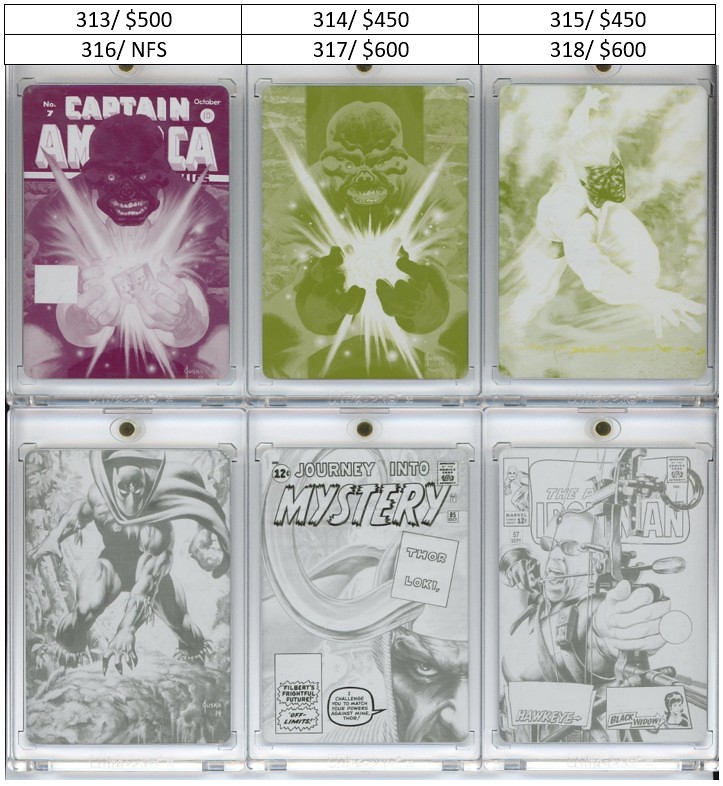This image is a color photograph of six comic book covers or trading cards, each encased in plastic protectors and displayed in a square format with two rows of three covers each. At the top left, there's a vibrant purple and white comic featuring Captain America standing beside an ominous alien figure who resembles Red Skull. This figure is holding a glowing, floating cube of energy. Directly next to it in the top row is the same comic book cover, but in striking green tones and without the Captain America text. To the far right of the top row is a different comic cover also in green shades, depicting a person climbing a rock wall.

In the bottom left corner, there's a monochromatic comic cover of what appears to be Black Panther, facing the viewer in grey tones. The center cover in the bottom row reads "Journey into Mystery" at the top, featuring Thor and Loki in a detailed black-and-white illustration. Finally, the bottom right cover shows a man ready to release an arrow from his bow, with "Hawkeye and Black Widow" text at the bottom. All the comics display pricing and numbering information, indicating they may be purchasable or collectible items, possibly NFTs, with prices ranging from $450 to $600. The entire collection exudes a mix of vivid color schemes, grayscale tones, and varying artistic styles, making for an eye-catching and diverse display.